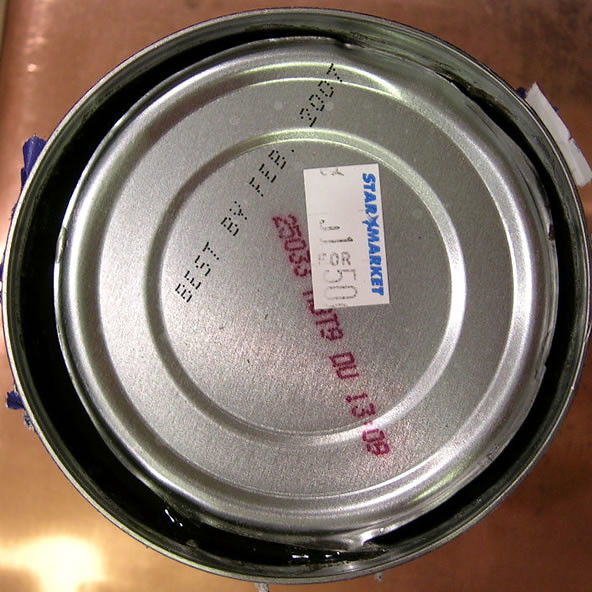A top-down view captures a can positioned against a metallic or copper-colored background, suggesting it may be placed on a metal table or kitchen stovetop. The can appears to be opened, indicated by the jagged edges around the perimeter where a can opener has cut. The interior of the can is mostly obscured by darkness, making its contents indistinguishable. The can’s exterior label is partially torn, revealing various pieces of information on the top.

Prominently displayed on the can's lid is a "Best By" date marked in black font, reading "February 2007." Adjacent to this is a partially visible red text, "25033," with the rest obscured by a label. Overlapping the red text is a white rectangular sticker from Star Market, featuring blue text. This sticker indicates a price, likely suggesting that the can was valued at 50 cents.